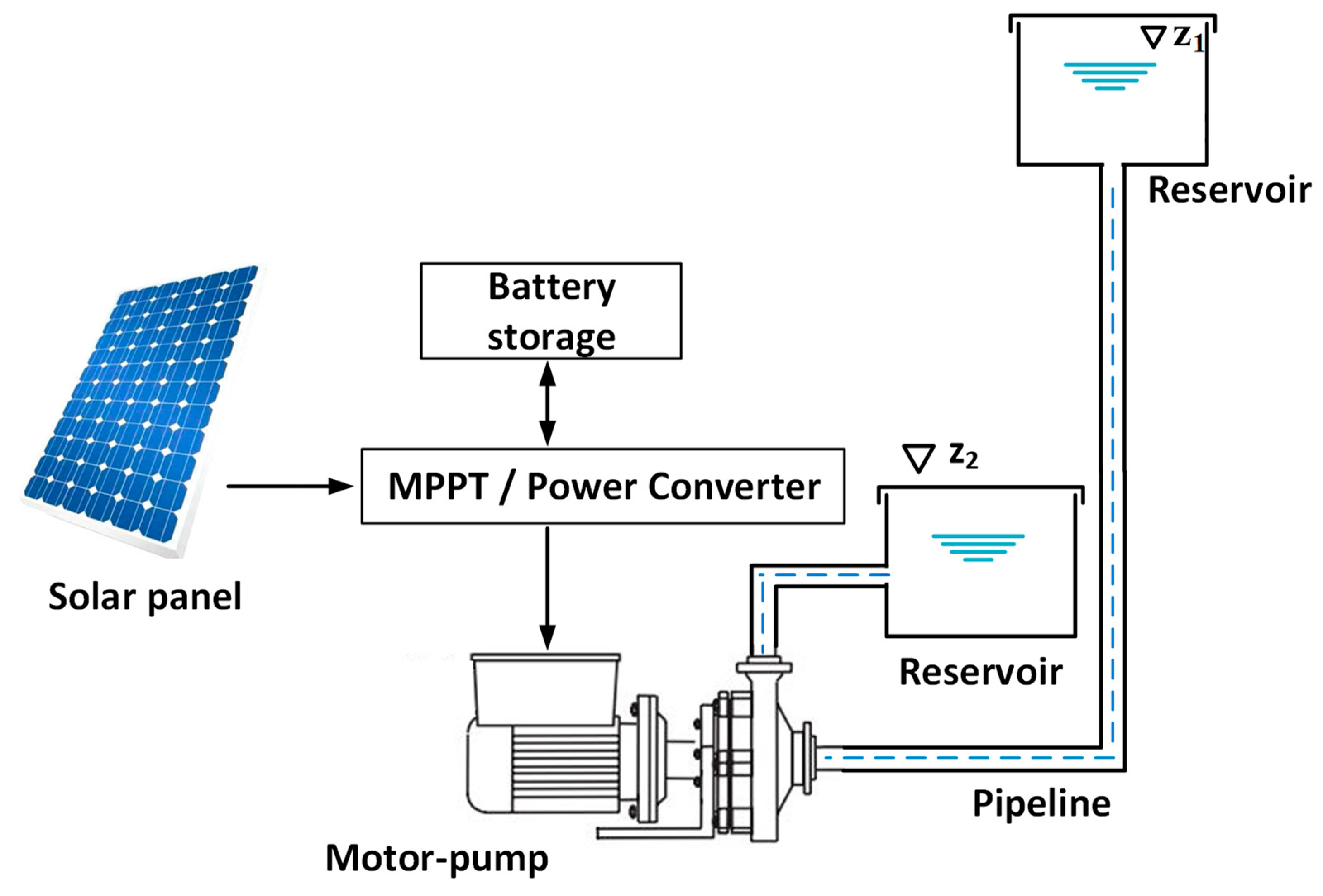The image is a detailed diagram of a solar-powered water pumping system, utilizing a blue and white color scheme with various text and arrows for explanation. In the left middle, a blue square with white dots represents a solar panel, labeled "Solar Panel." Arrows from the solar panel point to a box labeled "MPPT/Power Converter." Above this, another box labeled "Battery Storage" is linked via arrows. Below the converter, an arrow points to a "Motor Pump," illustrated with a black and white outline. The motor pump connects to a series of pipelines, directing flow to two reservoirs, each indicated with blue water levels and labeled "Reservoir." The image employs a combination of bright blue, darker blue, black, white, and light bluish-green colors. This engineering diagram elucidates the functional connectivity between solar panels, battery storage, power conversion, motor pumps, and water reservoirs.